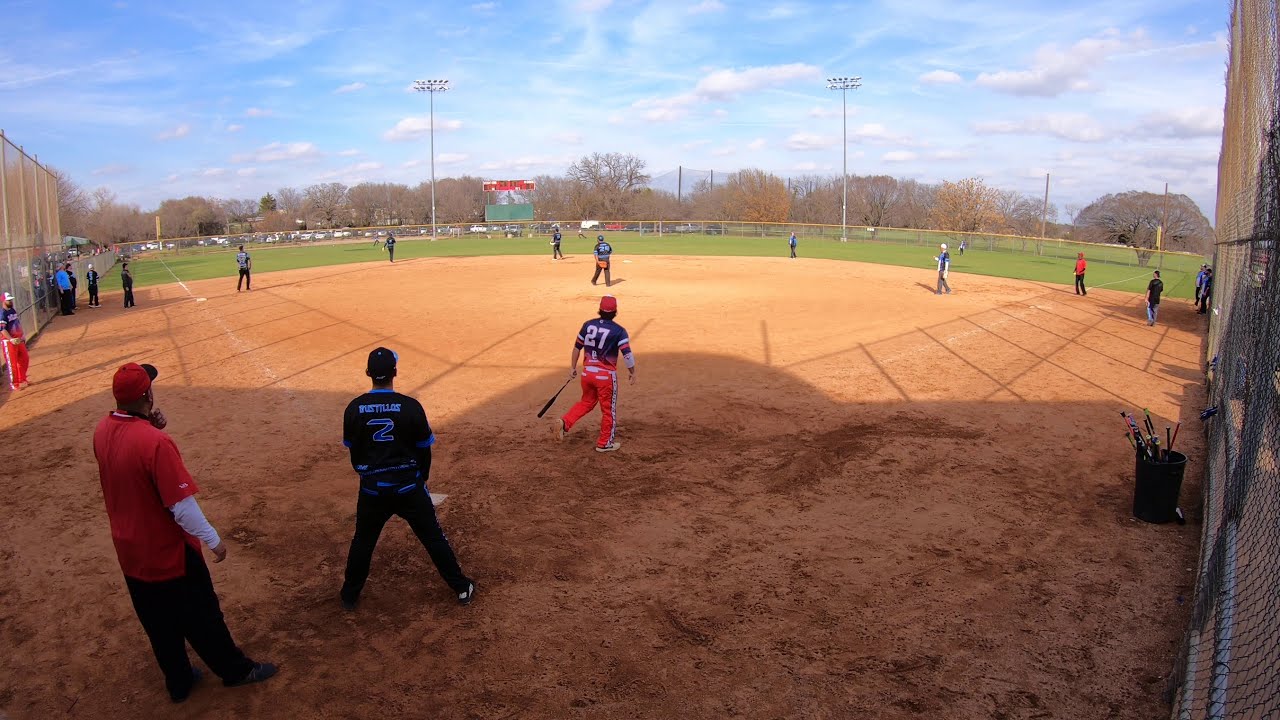The image captures a vibrant outdoor baseball game taking place in a stadium under a beautiful blue sky dotted with white, puffy clouds. The infield consists of tan and brown sandy dirt, with clearly marked white chalk lines indicating bases and various areas of play. White bases are scattered across the field, leading up to a boundary marked by a chain-link fence with a yellow top. Beyond the fence stand several dry, brown-colored trees, adding a natural backdrop. 

In the center far background, a green scoreboard is visible, above which sits an electronic white and red scoreboard. The field is populated by numerous players wearing diverse clothing, each in their positions. Closest to the camera stands a person wearing a red shirt, red hat, and black pants, likely a referee, directing the game. Nearby, a player is seen in a black and blue jersey, positioning himself for the next move. Another prominent figure is a player with the number two on his back, wearing a black t-shirt, black pants, and a black hat. Stadium lights tower over the boundary areas, casting their gaze over the field, ready for evening play. This detailed snapshot encapsulates the dynamic and lively essence of a baseball game under perfect weather conditions.